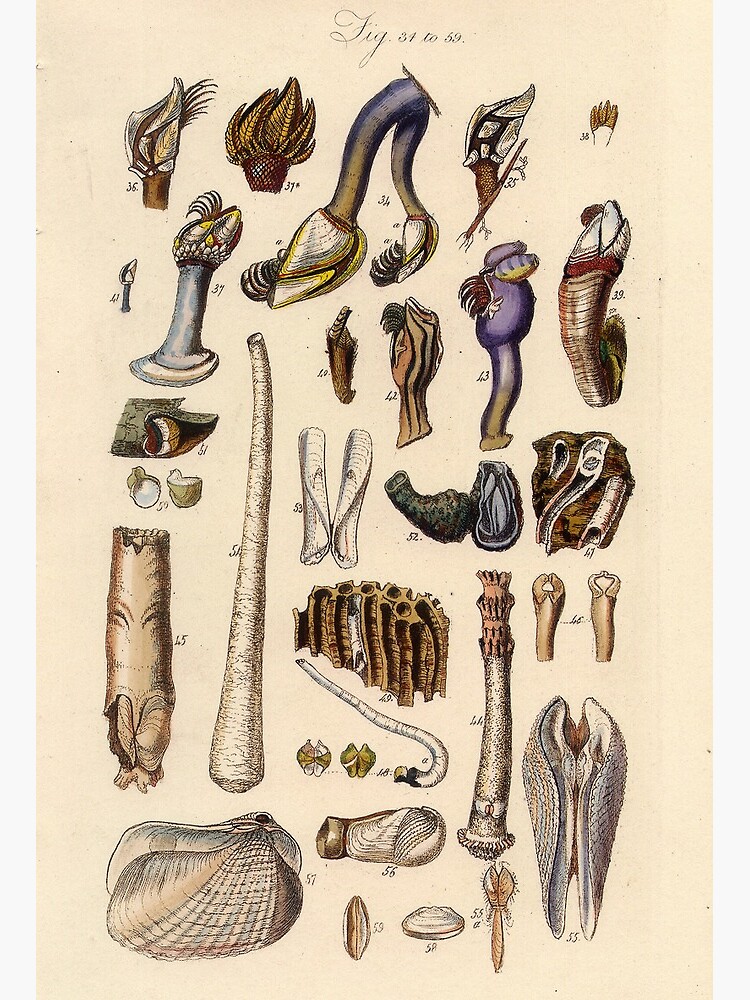This image appears to be an intricate study drawing, possibly an insert from an antique book, illustrating various sea life, primarily focusing on seashells and clams. The paper itself has a yellowish-beige tone, adding to its vintage feel. The illustration features around 50 hand-drawn objects, each uniquely numbered and annotated with cursive lettering at the top, indicating numbers "34 to 59." The objects are predominantly colored in shades of purple, yellow, and brown-gold, creating an organic and natural palette. The seashells come in diverse shapes and sizes—some fluted, some curvy, and others pointy, with lines and details giving them a lifelike appearance. Certain images resemble actual sea creatures more than shells, adding a sense of variety. Despite not being able to identify all objects precisely, the overall style and presentation suggest an old-fashioned, possibly educational purpose, focusing on the rich diversity of marine life.